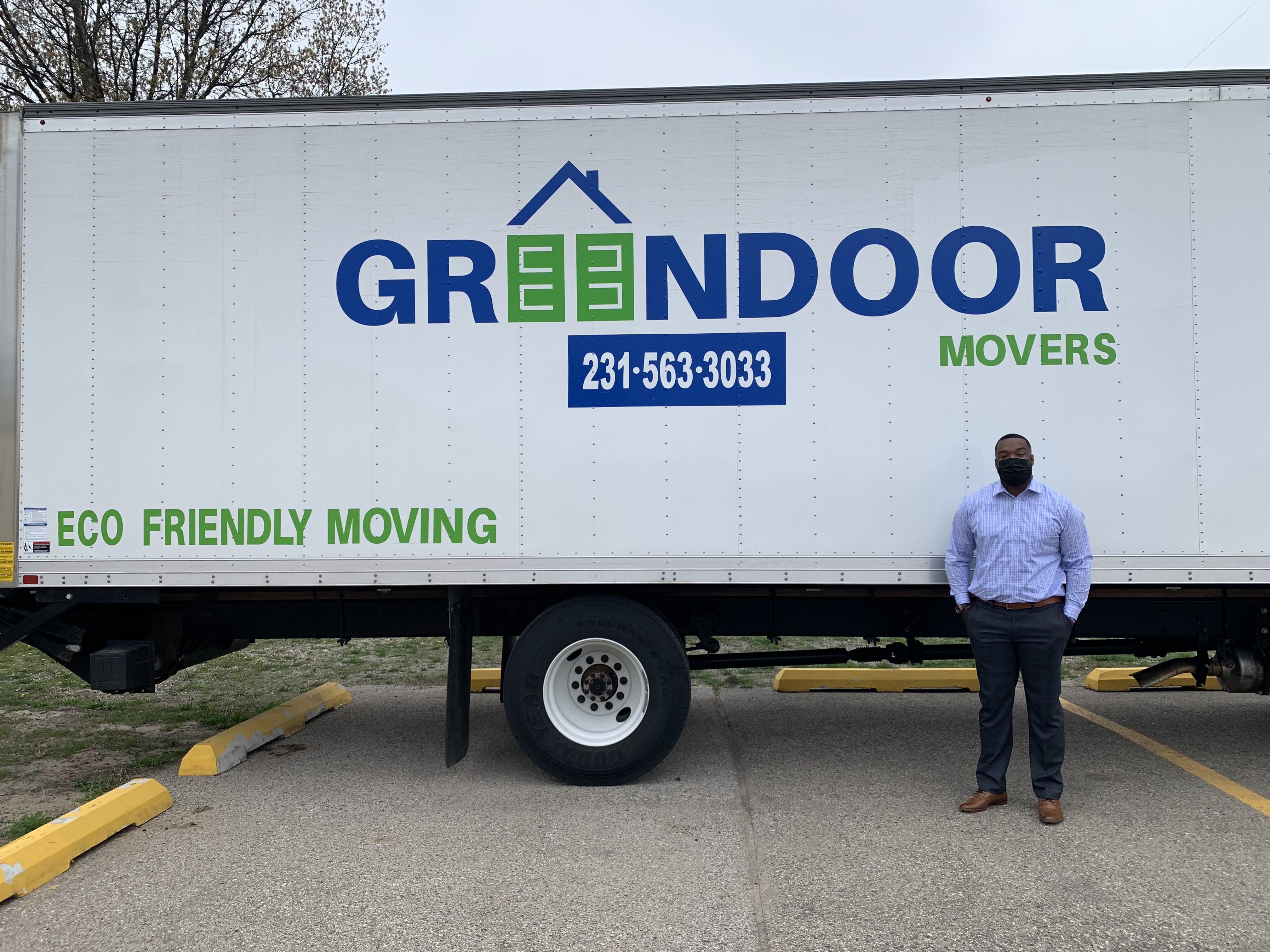This color photograph captures an African-American man standing in a parking lot on asphalt marked with yellow painted lines and curbs. He is dressed in a blue and white striped button-down shirt, dark gray dress pants, brown leather shoes, and a black face mask. He stands beside the prominently featured side of a large white box truck, positioned side profile. The truck's side panel displays "Green Door Movers" in blue and green lettering, with unique green square designs replacing the E's in "Green Door." Below the company name is a blue rectangle with the telephone number "231-563-3033" in white text. In the lower left corner of the truck's side, it states, "Eco-Friendly Moving" in green. The upper part of the image captures blue sky and tree branches, providing a natural backdrop to the urban parking lot scene.